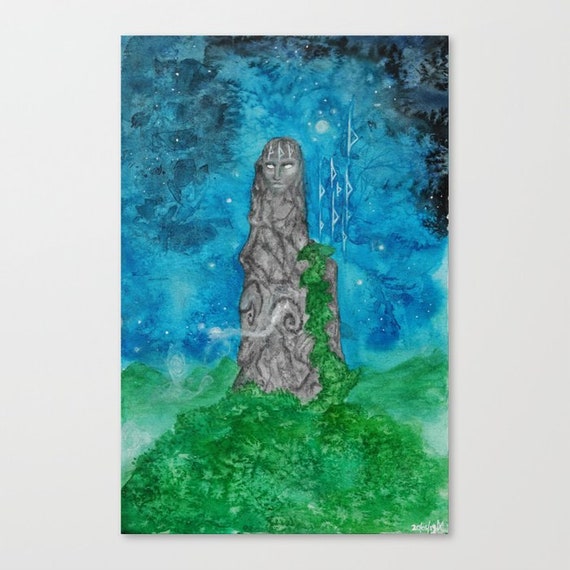The image is an illustrated drawing that appears to be set on a white background. In the center, it features a remarkably detailed stone statue of a person whose face is adorned with strange, glowing runes on the forehead. The statue, made of solid rock, portrays what might be a woman wearing a robe intricately designed with swirls, geometric shapes, and horned patterns along its lower end. Partially overgrown with ivy and foliage, the greenery climbs halfway up the statue and extends down to form a mound of grass at the base. The backdrop of the illustration depicts a nighttime sky, abundant with stars and overshadowed by clouds, rendered in varying shades of blue and black. To the right of the statue, additional runes are dispersed across the sky. Shadows suggesting the presence of trees add depth to the scene. The image also includes an indecipherable white signature in the bottom right corner, and the ethereal ambiance of the night sky is illuminated by a partial moon.